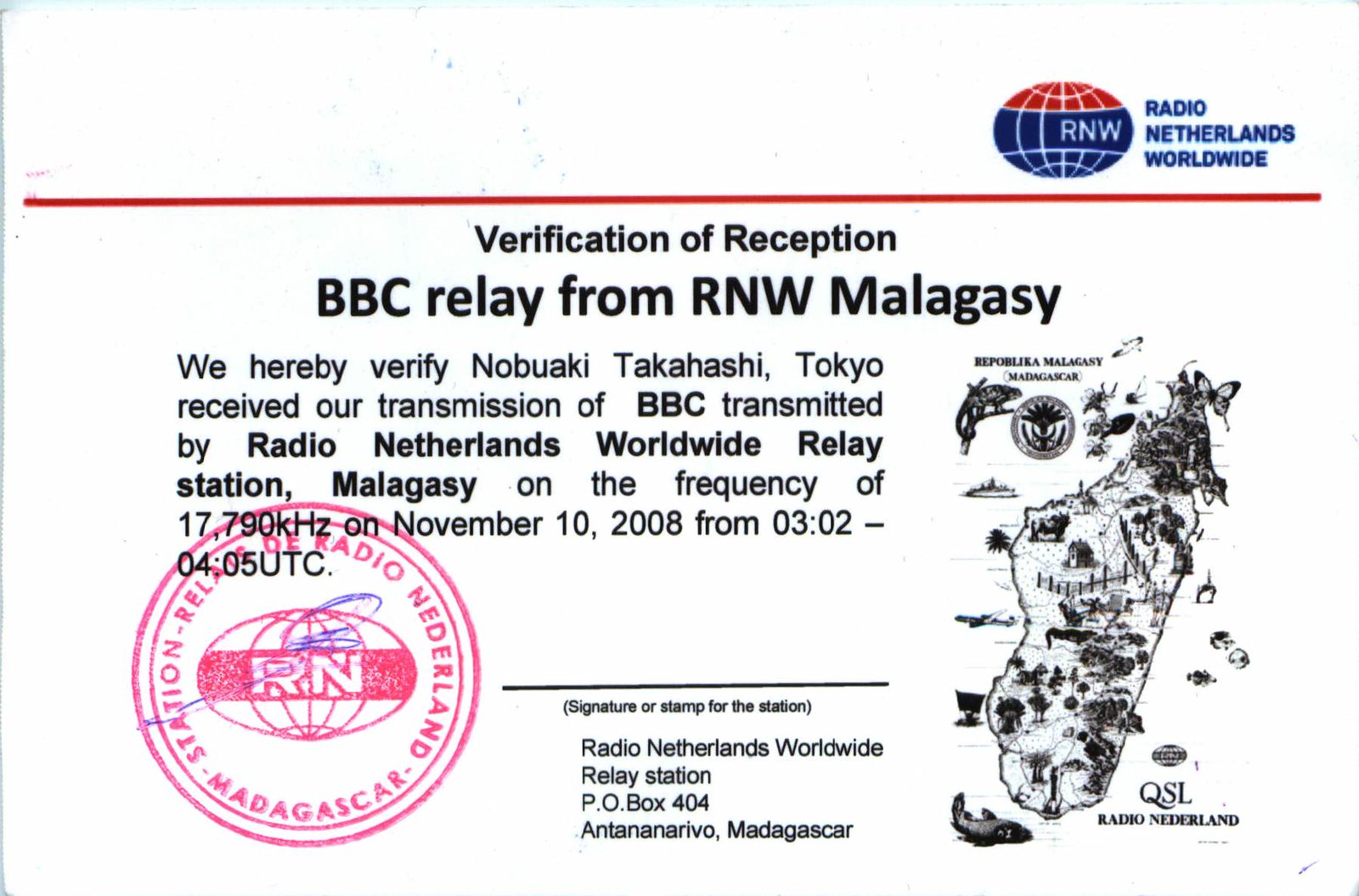The image depicts a QSL verification card from Radio Netherlands Worldwide. At the top right, the blue and red logo of Radio Netherlands Worldwide is prominently displayed, adjacent to a red horizontal bar. The card is titled "Verification of Reception: BBC Relay from RNW Malagasy." The detailed text on the card verifies that Nobuaki Takahashi from Tokyo received the first transmission of the BBC, relayed by Radio Netherlands Worldwide's station in Malagasy, on the frequency of 17,790 kHz on November 10, 2008, from 0302 to 0405 UTC. The bottom left corner features a red stamp from Radio Netherlands and additional address information, including the relay station's post office box in Antananarivo, Madagascar. The right-hand side of the card contains a map related to Radio Netherlands.